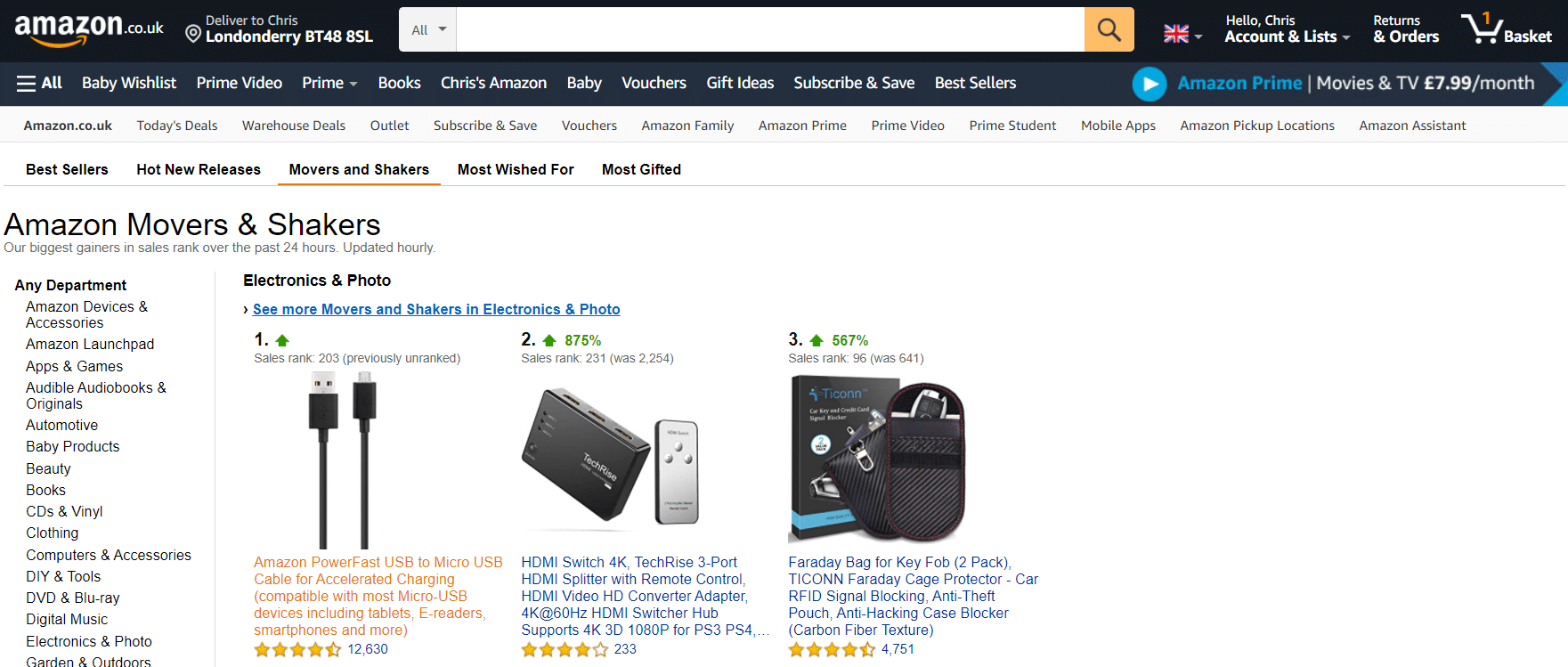Screenshot of the "Movers & Shakers" Section on Amazon.co.uk

This detailed color screenshot from a computer shows a user browsing the "Movers & Shakers" section on the Amazon.co.uk website. This section is indicated as the third of five selectable tabs, with adjacent tabs being "Bestsellers," "Hot New Releases," "Most Wished For," and "Most Gifted." The "Movers & Shakers" tab highlights the biggest gainers in sales rank over the past 24 hours, with updates occurring hourly.

The screenshot focuses on the "Electronics & Photo" category. The top three products in this category are:

1. **Amazon PowerFast USB to Micro USB Cable for Accelerated Charging** - This product holds the number one position in sales rank.
2. **HDMI Switch 4K TechRise 3 Port** - Ranked second in popularity.
3. **Faraday Bag for Key Fob 2-Pack** - Secured the third spot in sales rankings.

Each of these products has a customer rating between four and five stars. The interface also displays various page features and user-specific information. For example, it shows the delivery address as "Chris, Londonderry BT48 8SL," indicating the account owner's details. Additionally, there is a note that the user has an item in their shopping basket, although the specific item is not visible in the screenshot.